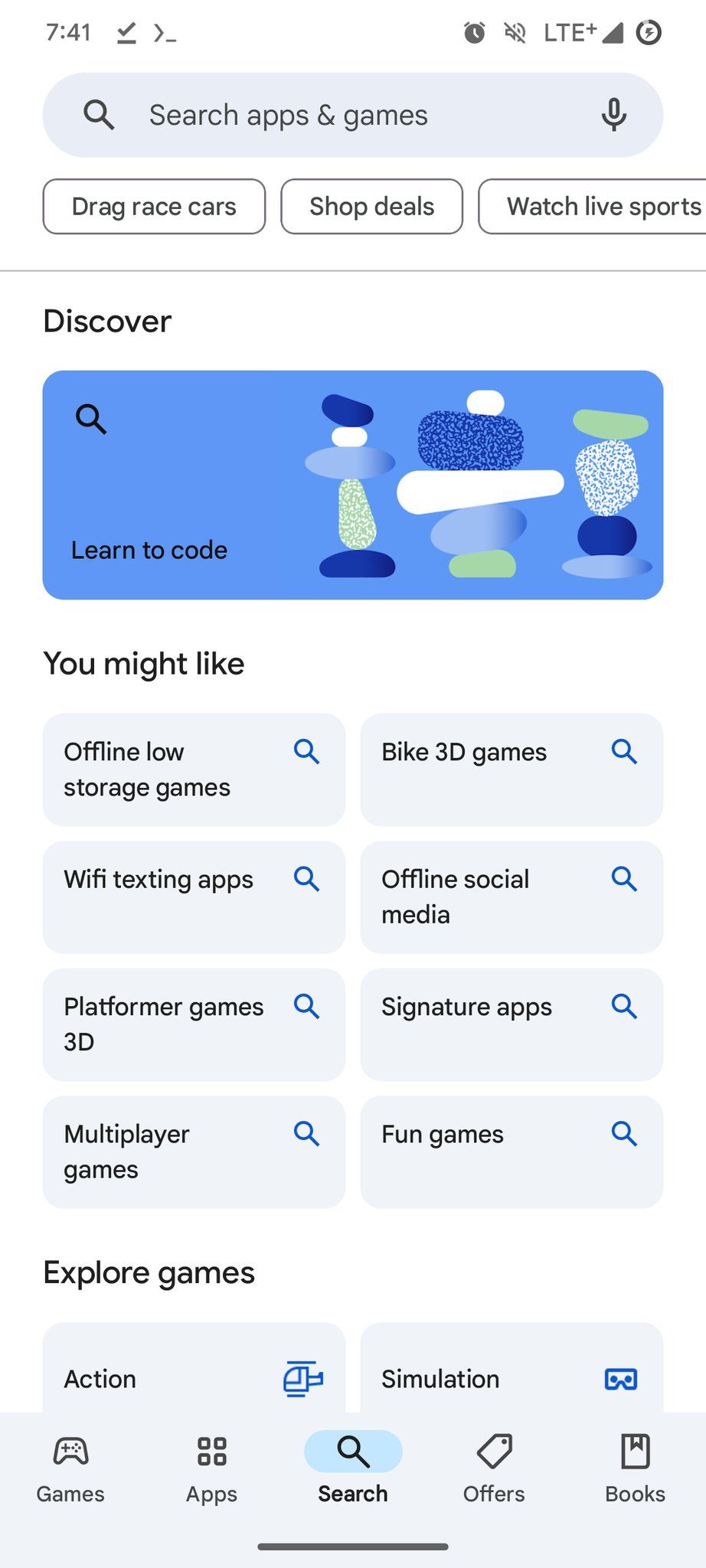This screenshot from a phone displays a user interface with a predominantly white background. At the top left corner, the time is shown as 7:41 AM, and there is no alarm set. The battery indicator is not visible. Below the time, a light gray oval encloses the text "Search apps and games."

Directly underneath this search bar, there are several quick access options: "Drag Race Cars," "Shop Deals," "Watch Live Sports." A thin light gray line separates these options from the rest of the content. 

In bold black and gold letters, the word "Discover" is prominently displayed. A light blue oval labeled "Learn to Code" follows this section. Further down, another header in black and gold letters reads "You Might Like," introducing various categorized options including "Offline Little Storage Games," "Bike 3D Games," "WiFi Texting Apps," "Offline Social Media," "Platformer Games," "3D," "Signature Apps," "Modifier Games," and "Fun Games."

Continuing downward, another section titled "Explore Games" in black and gold letters is visible, leading into categories like "Action" and "Simulation." The bottom of the page features a concluding gray line.